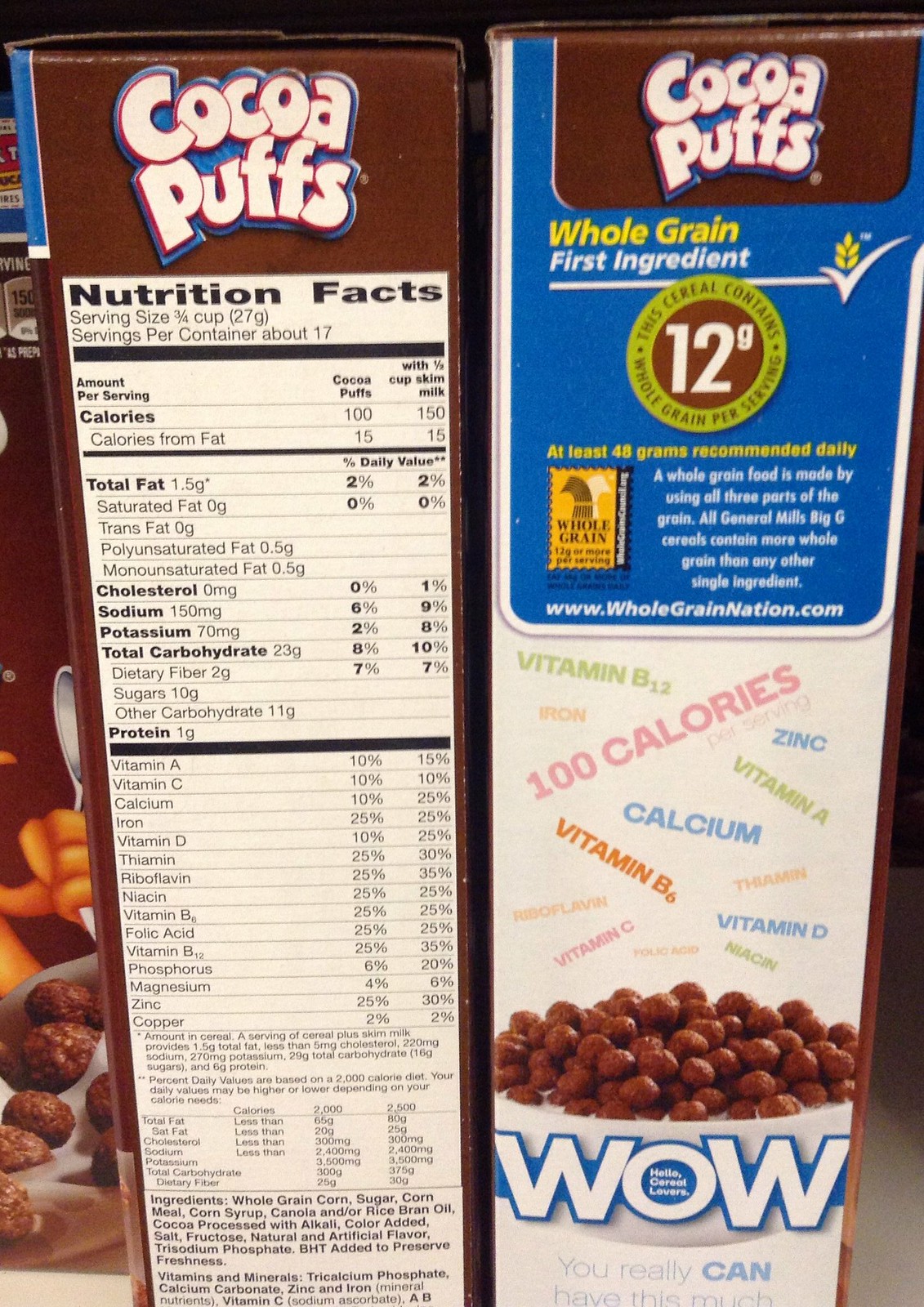The image showcases two Cocoa Puffs cereal boxes standing side-by-side, presenting their narrow edges to the viewer. The box on the left features detailed nutritional facts, starting with the prominent white "Cocoa Puffs" text at the top, followed by comprehensive information regarding calories, total fat, cholesterol, sodium, potassium, total carbohydrates, protein, and various vitamins. The right-hand box highlights notable features, also beginning with "Cocoa Puffs" in white text at the top. Beneath that, in a blue section, it emphasizes the whole grain content, stating "whole grain, first ingredient, at least 48 grams recommended daily," followed by another nutritional note. The lower part of the box displays a colorful advertisement-like segment mentioning specific vitamins (such as B12, A, B6, and iron) with a caloric content of 100 calories per serving. A vivid picture of a bowl filled with Cocoa Puffs and milk is positioned at the bottom, accompanied by the word "WOW!" in bold lettering. Additionally, a third box can be seen just barely peeking in from the far left, offering a partial view of its front side with a bowl of the cereal.